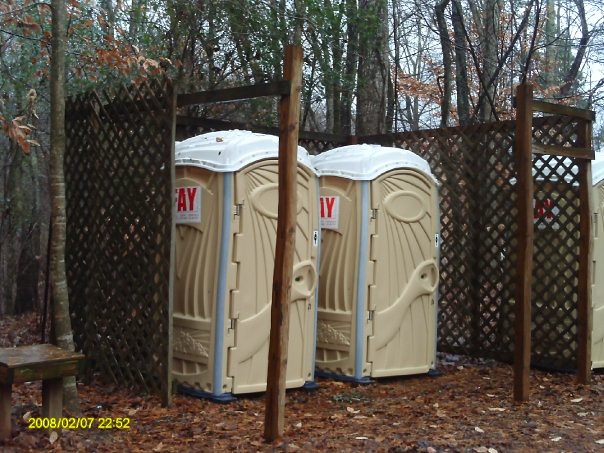This detailed color photograph, timestamped February 7th, 2008 at 22:52, depicts two tan port-a-potties positioned side-by-side within a partially enclosed structure. The port-a-potties, identical in design, feature gray corners, white roofs, and a relief scene on their fronts. The obscured company logo is visible in red letters against a white sign, displaying something ending in "AY."

The enclosure is constructed from wooden posts resembling debarked tree trunks, framed with two-by-fours, and covered in brown-stained latticework. This framework is open towards the viewer, allowing an unobstructed view of the two port-a-potties. The ground around them is covered in pine needles, bark, or mulch, indicative of a natural setting.

Though the focus is on the two port-a-potties, there is a third identical unit partially visible behind the latticework on the right-hand side. In the lower left-hand corner, a small flat wooden bench or table is present next to a slender tree trunk.

This image is set against a backdrop of deciduous trees, some leafless and others clinging to dead leaves, suggesting an autumnal scene. The timestamp and date are displayed in yellow text in the bottom left corner, marking this moment in time.